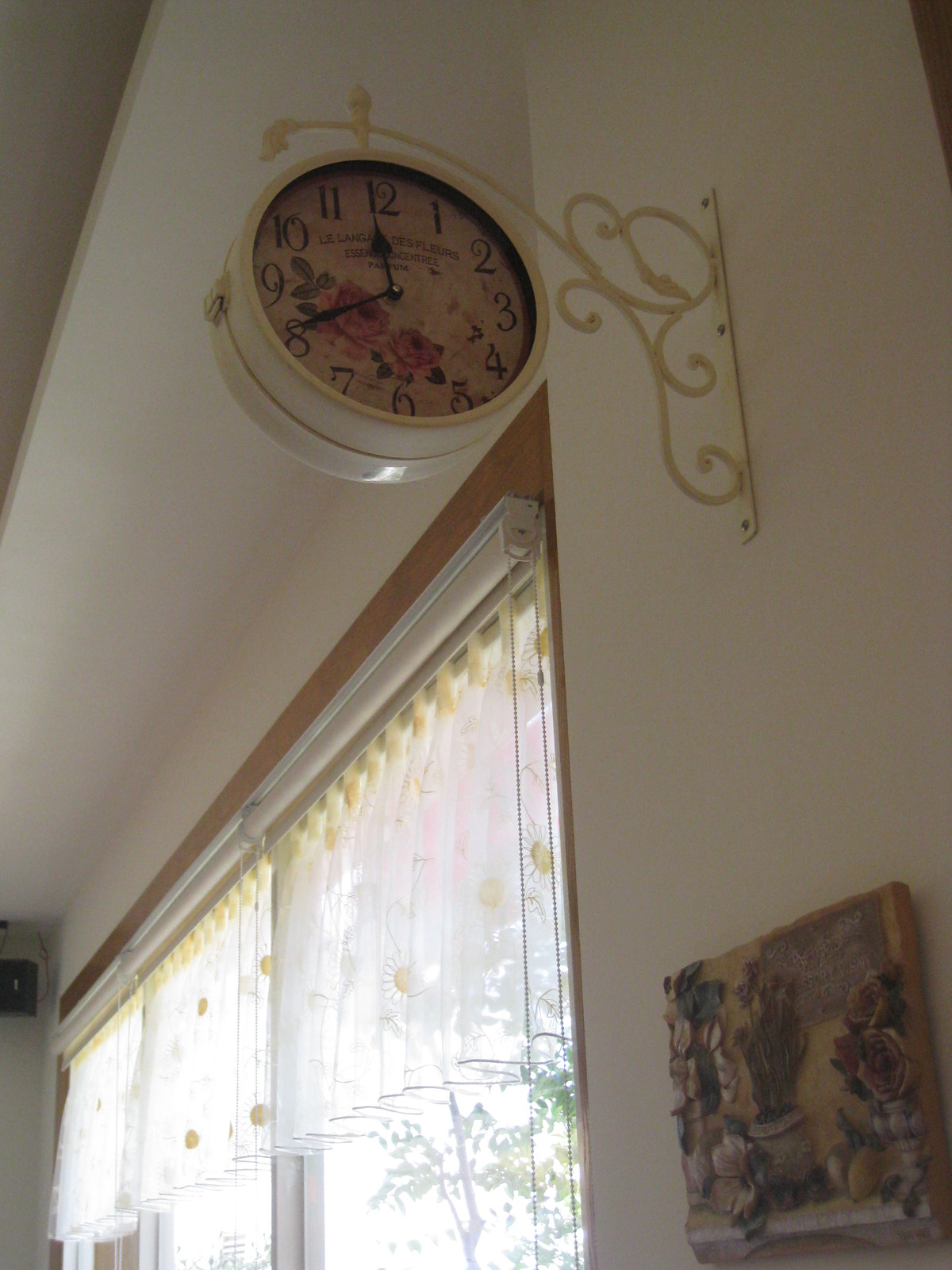The image captures a cozy interior setting, possibly a dining room or kitchen, with a vertically rectangular frame and dim lighting. The focal point is a large, ornate clock hanging on the right side of a cream-colored wall. The clock is held by an elegant cream-colored metal bracket that extends out from the wall, featuring intricate, wrought iron-style swirls. The clock itself has a beige background adorned with a delicate floral design, including pink roses on the face, and prominently displays large black numbers with two black hands. The smaller hand is positioned at the 12, and the larger hand is at the 8, with a visible seam and hinge, suggesting the clock may open.

Just below the clock, there is a decorative stone or ceramic piece featuring neutral-colored vases with an arrangement of flowers and plants. 

To the left of the clock, the wall transitions to a row of double windows that stretch from the central part of the frame. These windows are dressed in sheer curtains embellished with a daisy pattern—white petals with large yellow centers—and topped with a yellow trim. Bright daylight filters through the windows, illuminating the interior and providing a view of lush green trees outside.

The tan ceiling and the placement of a window beneath suggest a cozy, welcoming atmosphere typical of a lived-in home.